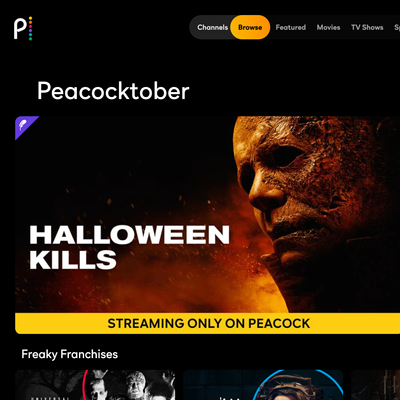Screenshot of a Promotional Advertisement on Peacock

The image is a promotional screenshot for "Halloween Kills," seemingly run by Peacock. The background is predominantly black. At the top left, the Peacock logo is visible, featuring a white lowercase "p" followed by five colorful dots in yellow, red, green, blue, and purple. 

On the right side of the image, several menu options are displayed: Channels, Browse, Featured, Movies, TV Shows. The 'Browse' button is distinguished by an orange circle indicating it has been selected, while the other buttons are grayed out.

Positioned slightly to the left, the text "PeacockTover" appears in a white font. Below this text is an ominous photo of Michael Myers, the iconic character from the Halloween film series, situated on the right side of the page. "Halloween Kills" is boldly written in white font on the left side. Directly beneath this in a yellow text box, it reads "Streaming only on Peacock." Further below, the image teases other horror films under the heading "Freaky Franchises," with partial images of two more movie posters, although the faces are cut off and not fully visible.